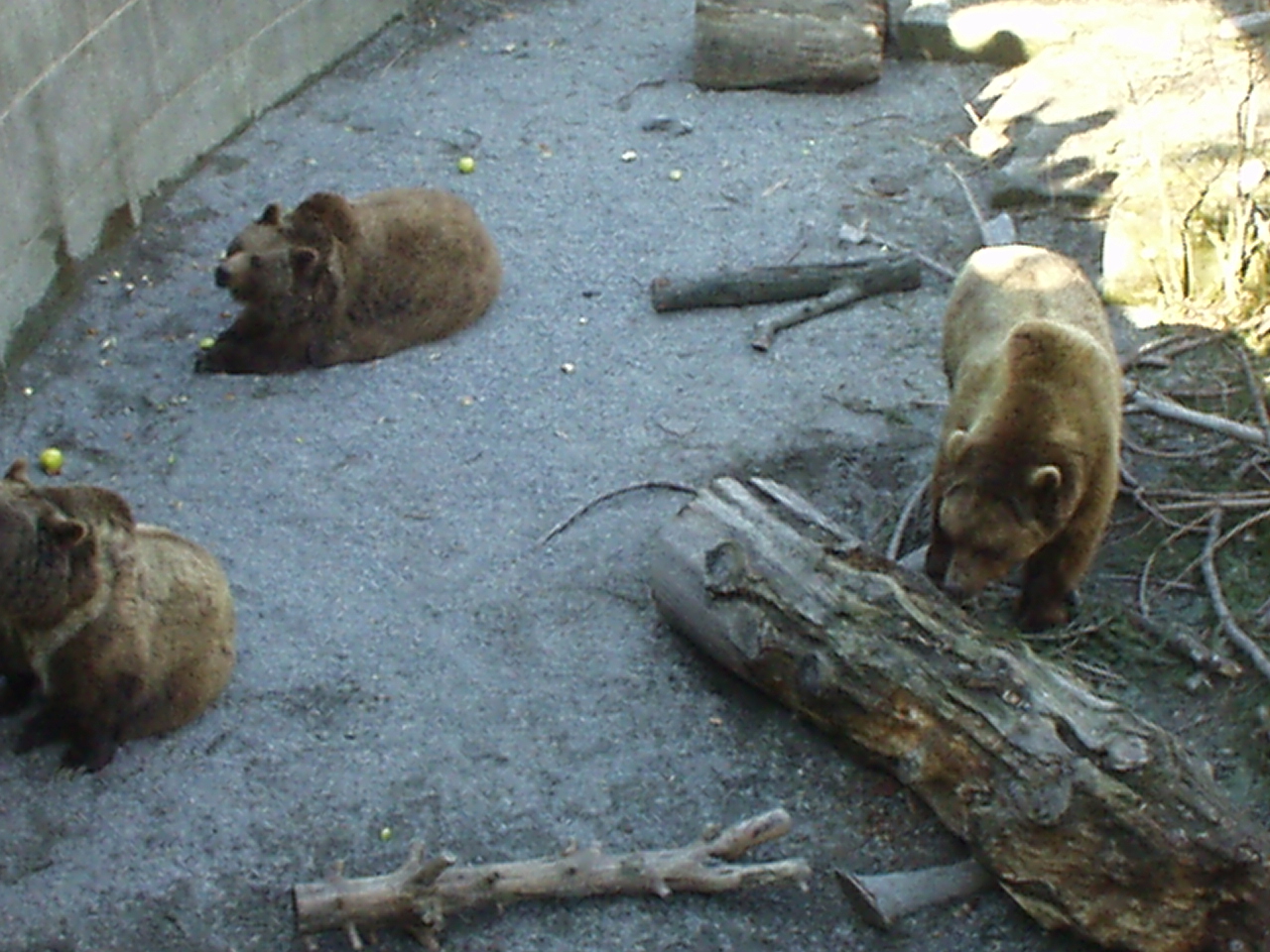The image depicts a somewhat grainy photograph of an enclosure featuring three brown bears on a gray, gravelly ground, interspersed with scattered logs and branches. One bear is laying down, another is sitting, and the third is standing, sniffing a decayed log in the lower right corner. Green apples or some type of fruit are strewn around the enclosure near the bears. The upper left of the image shows a cement wall, which likely serves as a barricade, suggesting the setting is a zoo. In the background, the upper right corner is illuminated by sunlight, highlighting some grass, twigs, and branches. The shadows of three or four spectators are cast within this sunlit area, indicating they are observing the bears from behind the barricade.